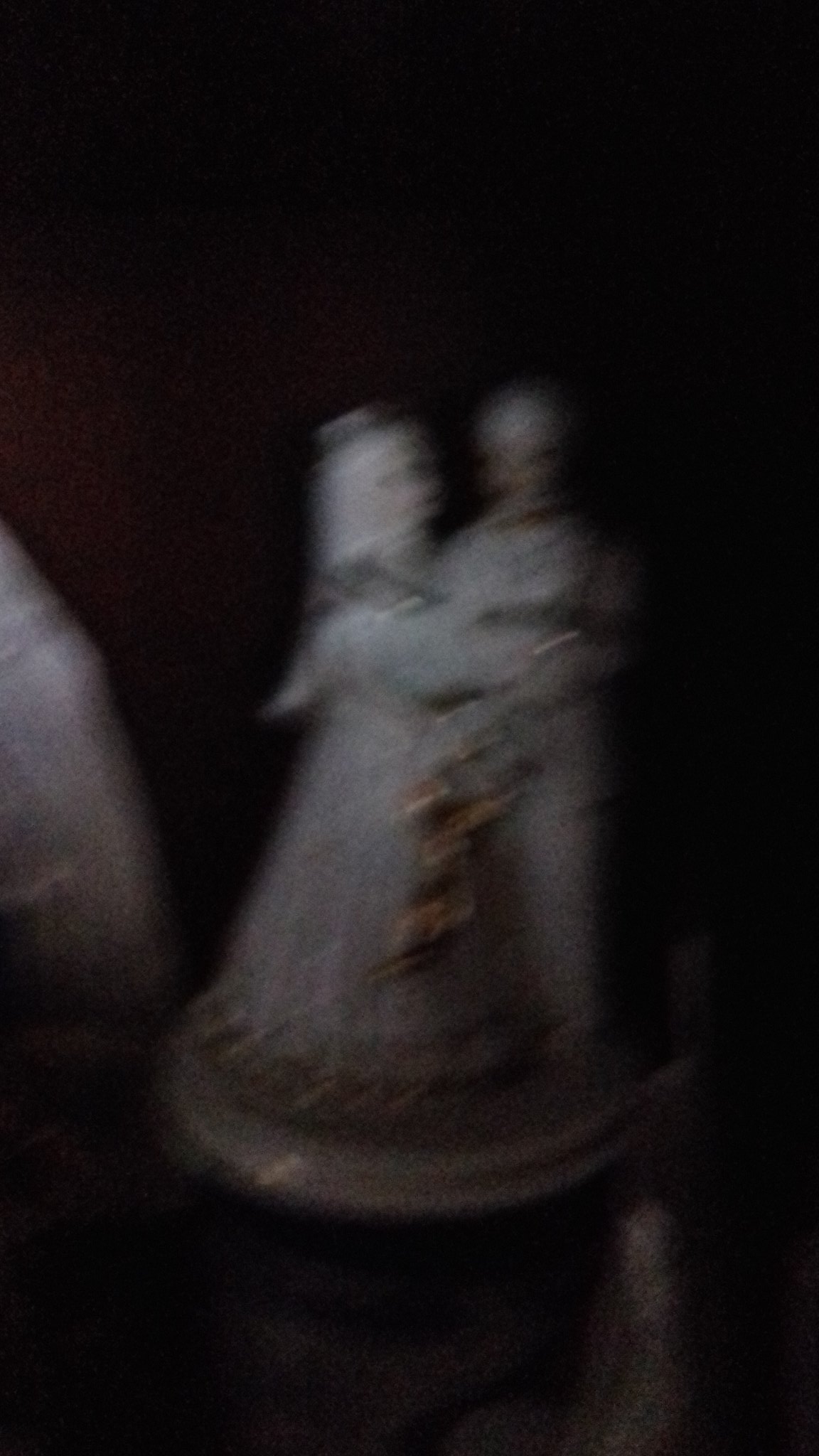The image displays a blurred scene of an ornament featuring a man and a lady engaged in a dance. Both figures are adorned in white attire; the lady is elegantly dressed in a long, flowing gown with gold trim at the hemline and appears to be wearing a hat. Her male partner is outfitted in a suit with trousers. They are depicted holding arms and performing a circular dance. The base of the ornament is semi-circular, enhancing the dynamic nature of their movement. This could either represent a dance or a wedding scene. In the background, there appears to be another indistinct ornament, with a white shape protruding from it, though its details are not clear. Both ornaments rest on a dark table, contributing to the overall blurry quality of the image.